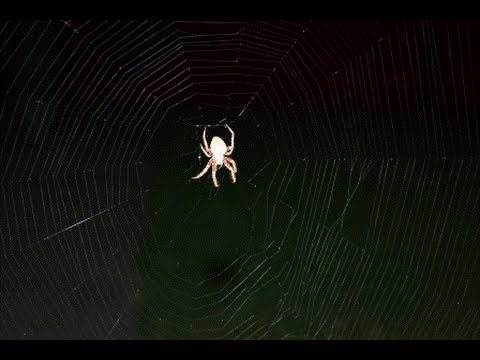A nighttime outdoor photograph features a large, circular spider web taking up most of the frame. At the center of the web, slightly to the left, hangs a prominent spider. The spider's abdomen is very white, reflecting the light, while its legs are a light sandy brown color with some yellowish hues. The spider is poised in the web, which is sparse near its body but becomes increasingly concentrated and detailed toward the edges. Notably, there is some damage and gaps in the web, particularly on the middle right side. The background is dark, with a gradient of black at the top and green at the bottom, suggesting a grass-covered area possibly between two trees. There are no insects caught in the web, and the whole scene is subtly framed by thin black borders at the top and bottom of the image.